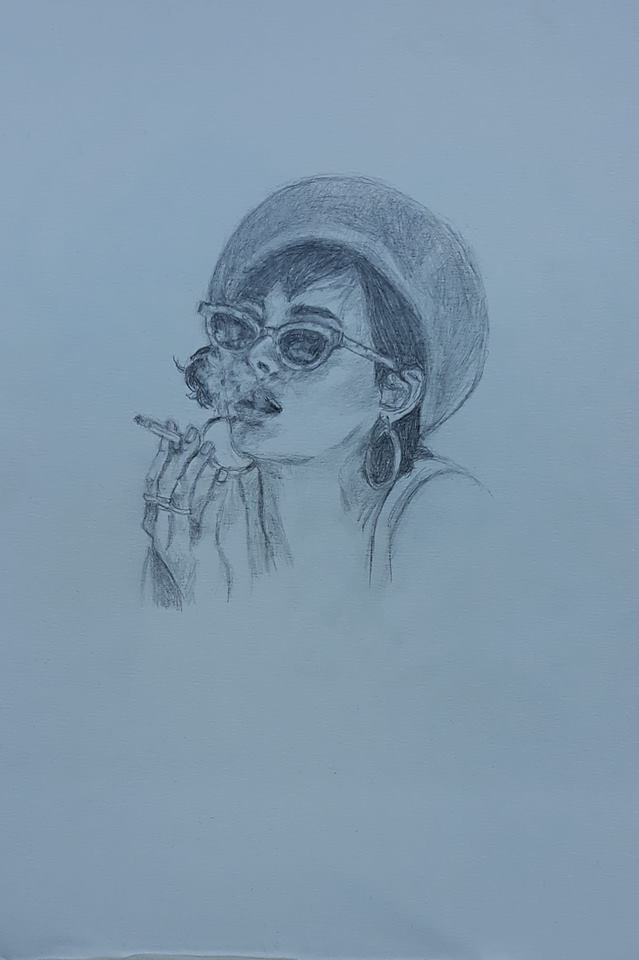This impressive pencil drawing, meticulously sketched on a light blue or gray sheet of paper, portrays a classically cool woman in a strikingly detailed portrait. With shoulder-length dark hair peeking out from beneath a stylish hat that resembles a large beret, she gazes to the right, exhaling smoke from a cigarette held in her right hand. Her hand, adorned with rings on the index, middle, and ring fingers, elegantly holds the cigarette that needs to be ashed. The woman sports large hoop earrings and chic cat-eye sunglasses, adding to her effortlessly cool demeanor. The precision in shading and intricate details, from her thick eyebrows to the contours of her face, makes this artwork extraordinarily impressive.